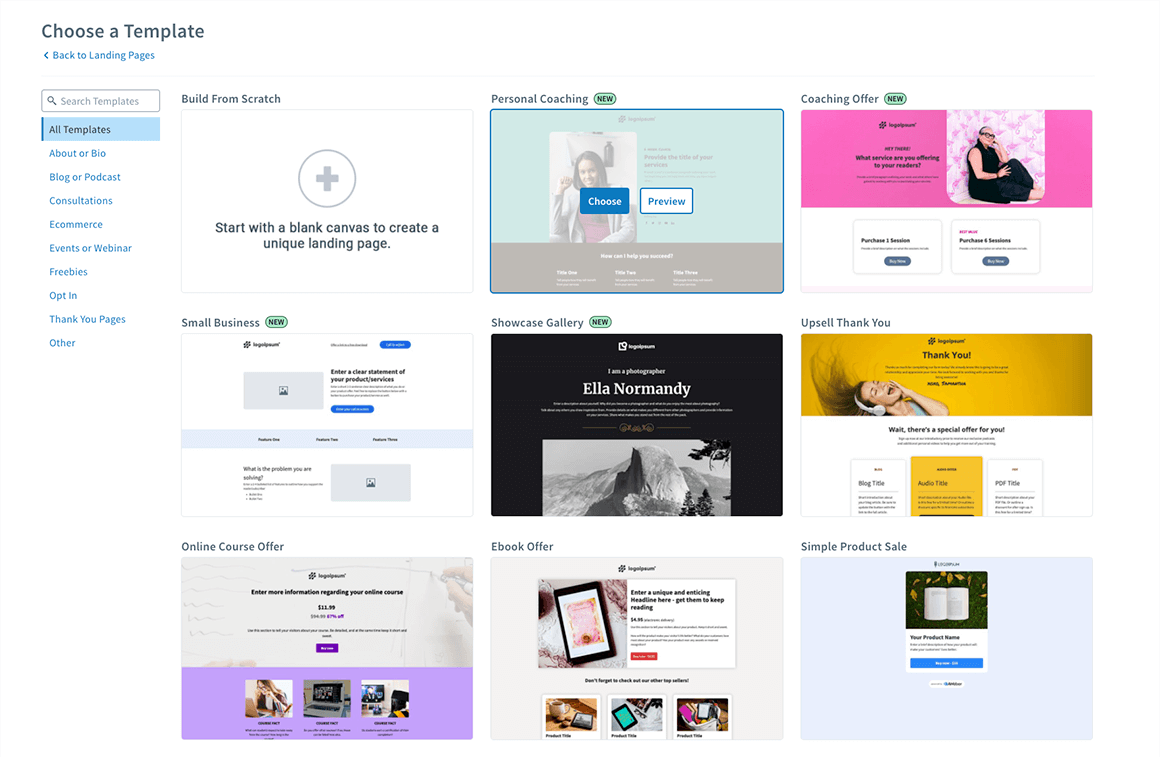The image showcases a selection of website templates on a webpage. 

- In the top-left corner, the header reads "Choose a Template." 
- An arrow pointing to the left with the text "Back to Landing Pages" is displayed beneath the header. 
- Directly below, a search box contains the placeholder text "Search Templates."
- The "All Templates" category is highlighted.

Below the header, several template options are presented:

1. **Build from Scratch**:
   - This option features a blank rectangle with a white background containing a circle with a plus sign in the center. The accompanying text reads, "Start with a blank canvas to create a unique landing page."

2. **Personal Coaching**:
   - This template is shown as a rectangle with a blue background transitioning to gray at the bottom. 
   - It features a photo of a woman and the text "Choose and Preview" overlays the image.

3. **Coaching Offer**:
   - This template is divided into two sections: a pink background on the top half and a white background on the bottom half, also showcasing a photo of a woman.

Further below are additional template options:

- **Small Business**:
  - The template rectangle includes a prompt to "Enter a clear statement of your product's services. What is the problem you are solving?"

- **Showcase Gallery**:
  - Designed for a photography website, this template presents a black background.

- **Upsell Thank You**:
  - Provides another example of a template design.

Lastly, three more template examples are listed:

1. **Online Course Offer**
2. **E-book Offer**
3. **Simple Product Sale**

This detailed display provides various template options for different needs and preferences, catering to the creation of unique and tailored landing pages.